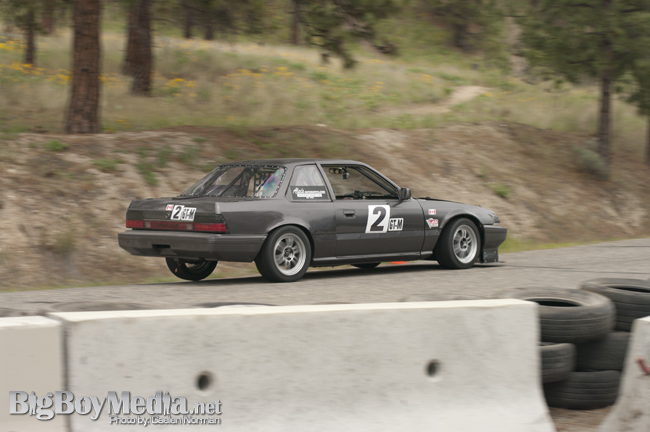This photograph captures a dark gray, two-door sedan with the number two and "GT-M" insignia on its side, indicating its possible use as a race car. The car is parked on a blacktop road, likely part of a race track, given the presence of concrete barriers and stacks of protective rubber tires nearby. The vehicle features black sportish wheels and standard hubcaps, with the windows rolled down, exposing a roll cage netting inside. In the backdrop, a scenic landscape unfolds, showcasing a meadow with trees, yellow flowers, and a winding footpath. The bottom left corner of the image credits the photographer, Galen Norman, through a watermark that reads "bigboymedia.net."